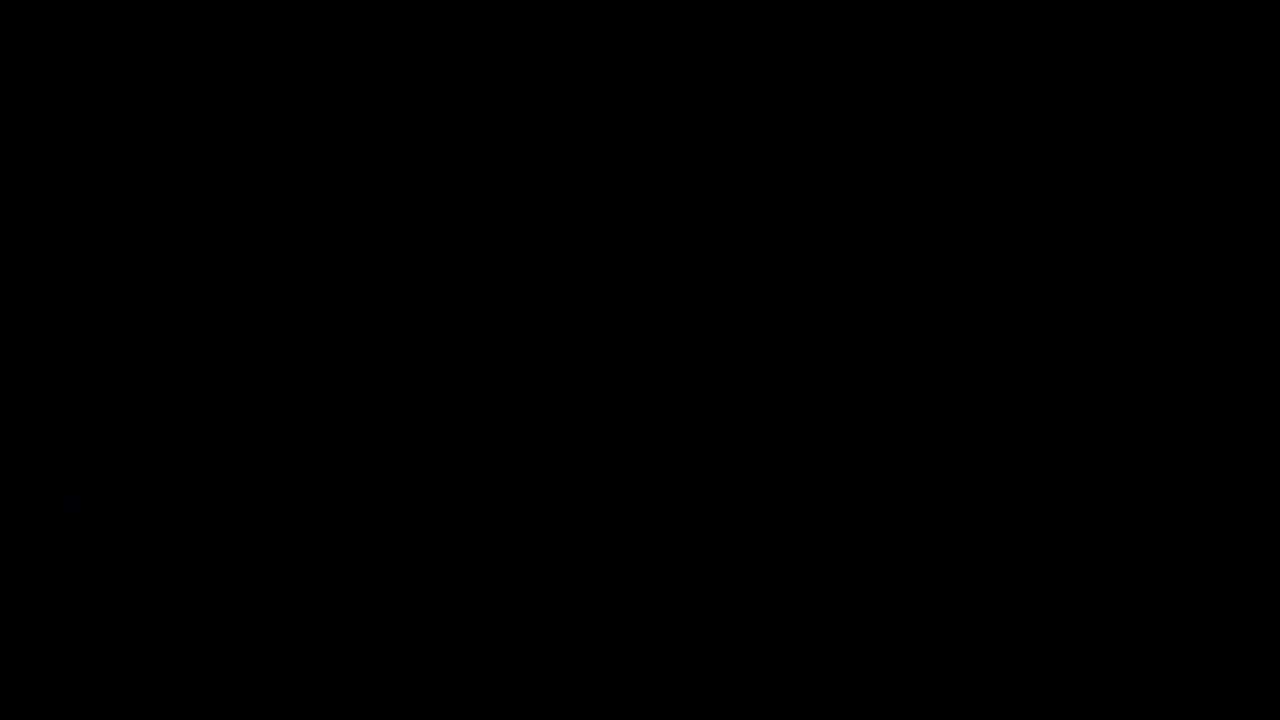The image is a large, solid black rectangle, longer than it is tall, with sharp, well-defined corners against a white background. It is completely devoid of any features, details, or gradations of color—just pure black throughout. There are no people, objects, words, or any identifiable elements in the image, making it unclear whether this is a photo taken with the lens cap on or a deliberate depiction of blackness. Its uniform and consistent color lends a definite separation from the surrounding white space, emphasizing the stark contrast. This complete absence of imagery might suggest a loading error or an intentional void, rendering it a pitch-black screen.